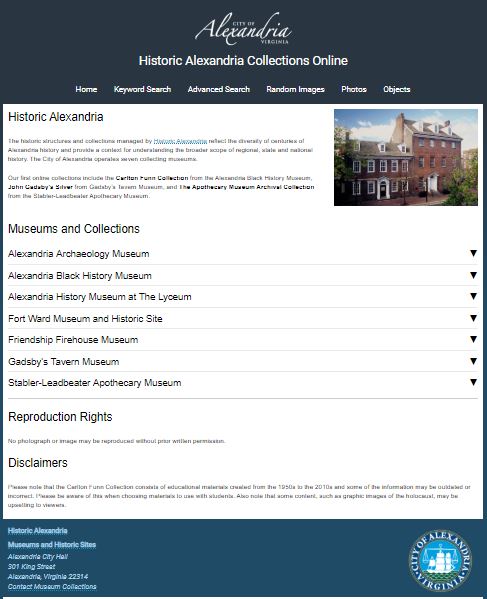This image showcases the City of Alexandria, Virginia's Historic Alexandria Collections Online website. The top of the webpage features a banner in a deep blue or slate gray color, with white font displaying options such as "Home," "Keyword Search," "Advanced Search," "Random Images," "Photos," and "Objects." Below the banner, on the left side, the header "Historic Alexandria" stands out against the white background. 

Below the header, two paragraphs provide some introductory information, though the text is not easily readable. Further down on the left side, there's a list of museums and collections including:

- Museums and Collections
- Alexandria Archaeology Museum
- Alexandria Black History Museum
- Alexandria History Museum at the Lyceum
- Fort Ward Museum and Historic Site
- Friendship Firehouse Museum
- Gadsby's Tavern Museum
- Stabler-Leadbeater Apothecary Museum

Following the list, a line separates additional sections containing "Reproduction Rights" and "Disclaimers," though the text is difficult to decipher. 

To the right of the museums list, there's a pull-down menu that allows users to explore further options on the site.

At the bottom of the page, a teal line provides contact information for the Alexandria Museums and Historic Sites, located at Alexandria City Hall, 901 King Street, Alexandria, Virginia 22314. It also includes information on contacting museum collections.